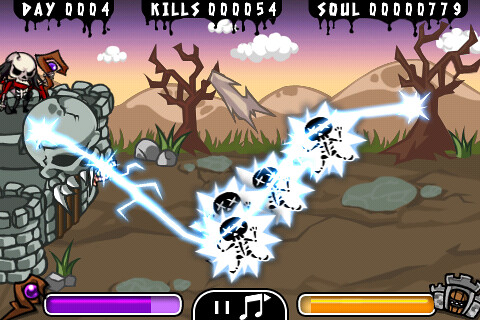This is a color screenshot of a retro-style platform video game, characterized by its airbrushed, simplistic art style. Dominating the left side of the image is a menacing stone castle topped with a large skull that emits a lightning bolt from the back of its head. This bolt interacts with four skeletons, possibly depicting a single character being electrocuted or sequential images of the character moving into the background. The lightning extends further, creating a dramatic effect as it reaches a distant tree. At the top of the image, game statistics are displayed: "Day: 0004," "Kills: 000054," and "Soul: 00000779." Below these stats, a purple and a yellow graph are visible, alongside a central section of text, beneath which are a pause button and a musical note icon. The vivid color palette includes purples, pinks, browns, greens, and grays, enhancing the visual appeal and nostalgic feel of the scene.